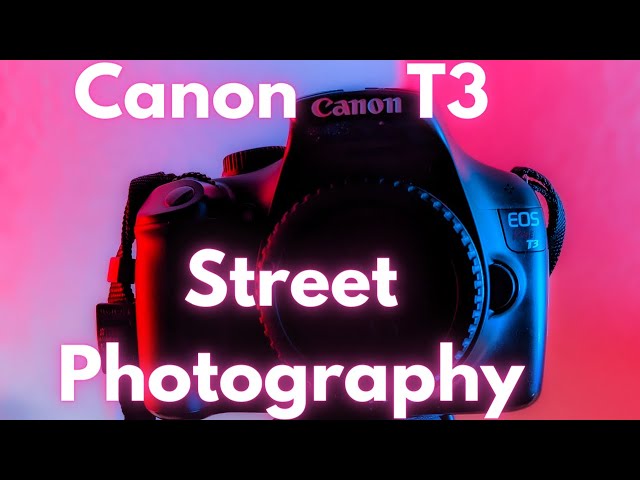The image depicts a black Canon DSLR camera, placed against a vibrant pink and blue gradient background that gives off a neon aesthetic. The photograph features strong letterboxing with black strips across the top and bottom, providing a clear frame for the subject. The camera itself is bathed in colored lighting, with a faint red light illuminating its right side and a blue light accenting its left, casting deep, contrasting shadows. The prominent text across the image reads "Canon T3" at the top, with "Street Photography" boldly positioned in front of the camera in large white font. Despite the dramatic lighting and vivid colors, the intricate details of the camera remain obscured by the shadows and highlights, emphasizing the artistic, almost abstract representation of the device.